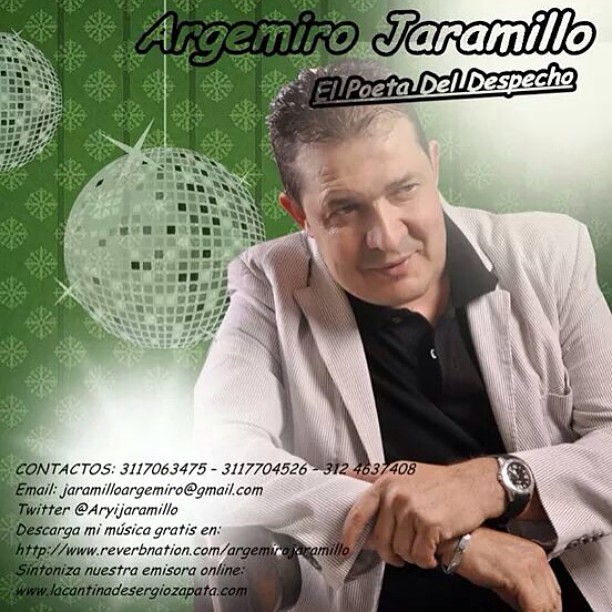The promotional image showcases a seated Caucasian man with slicked-back black hair, wearing a light gray or cream-colored jacket over a black button-topped polo shirt. He appears poised, with one hand clasping the wrist of his other arm, and he adorns a black watch. The man gazes off to the right, while the background features a graphic design element including a green curtain with two-dimensional white snowflake patterns, and two disco balls - one prominently centered and another partially cropped at the top left. At the top of the image, bold text reads “Argemiro Jaramillo, El Poeta del Despecho,” and the bottom left corner contains his contact information, including phone numbers, an email address (jamarioargemio@gmail.com), Twitter handle (@arijaramio), and two websites (http://www.reverbnation.com/argemirojaramio and www.lacanitadescargiosapata.com). The overall aesthetic blends retro graphics with modern promotional elements, illuminated by artificial lighting effects.